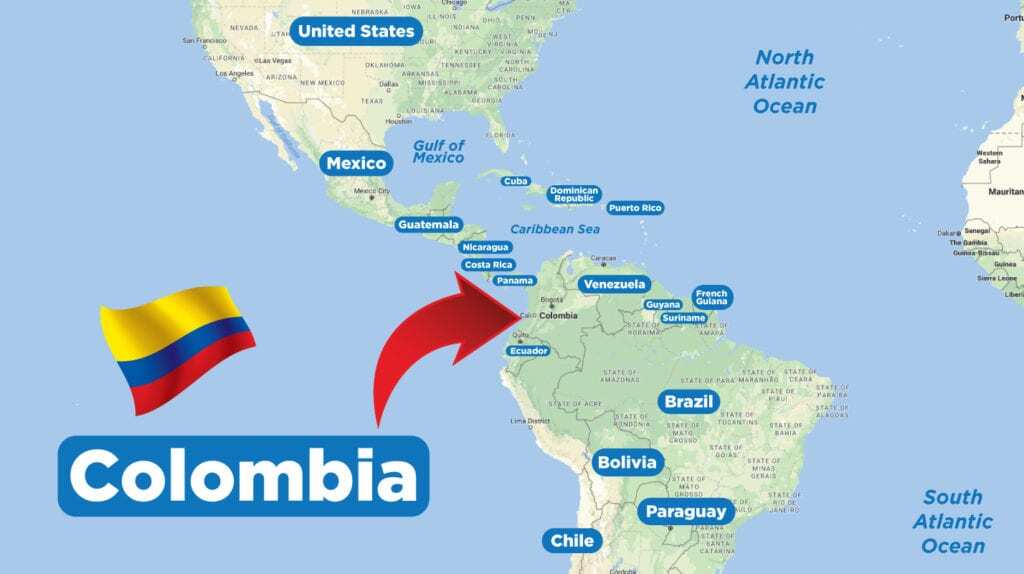This image is a detailed map highlighting significant parts of the Americas, including most of the United States, all of Mexico, and the majority of South America. The focal point of the map is Colombia, indicated by a prominent, large red arrow pointing directly at the country. Below the arrow, a sizeable blue bar with white text spells out "Colombia," accompanied by the Colombian flag, which appears to be waving in the air. This visual highlight is overlaid on the ocean to the left side of the map. In addition to Colombia, other major countries are labeled with similar blue ovals bearing white text, though none are as prominently featured as Colombia. The map features light blue oceans contrasting with green landmasses in varying shades. The upper portion of the map showcases the United States, while the southern section includes much of South America, ending around the regions of Chile and Paraguay.